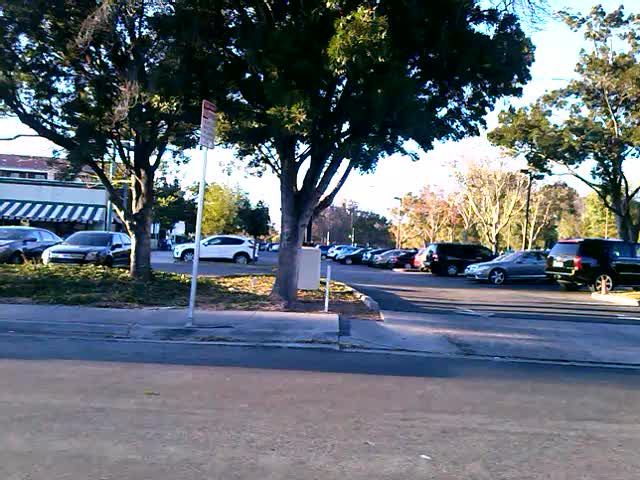Captured on a sunny day, this image showcases a bustling parking lot of a business viewed from across the street. The road in the foreground, made of asphalt, features visible arrows guiding traffic into and out of the parking lot. Numerous cars are parked in neat rows within the lot. 

Dominating the scene beside the road, a large tree stands tall in a grassy area, flanked by two smaller trees planted close to the entrance in a landscaped strip along the sidewalk. The landscaping includes an abundance of low, green plants that add to the greenery. A line of trees runs parallel to the parked cars on the right side of the lot, providing a touch of nature amidst the vehicles.

The sky above is a clear, vibrant blue, setting a perfect backdrop for the scene. On the left, a two-story building stands prominent, with its first level adorned by a green and white striped canopy extending outward, possibly marking the entrance to a business establishment. The overall atmosphere is bright and inviting, capturing a typical day at this location.